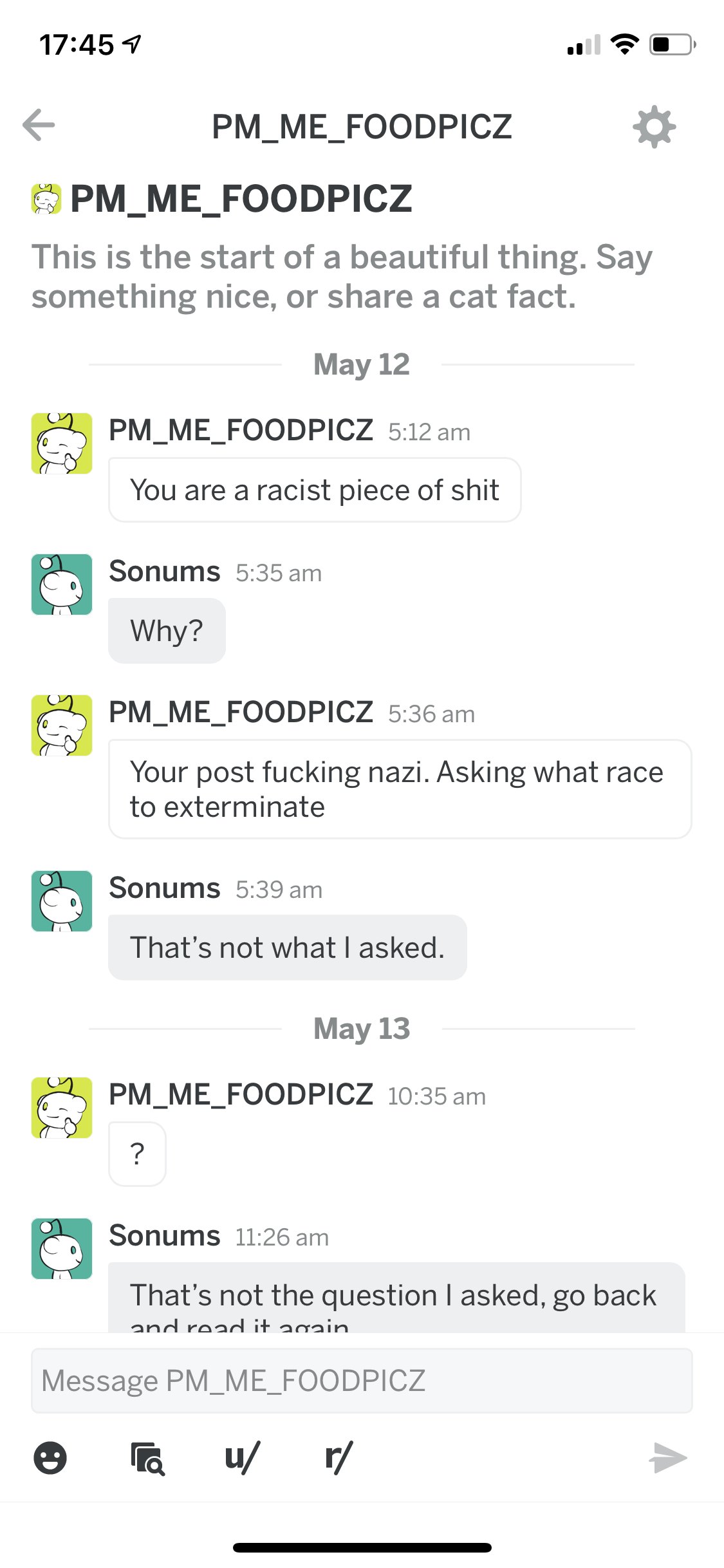In the image, there's a sequence of Reddit chat messages displayed against a white background. The initial message is from the user "pm_me_food_pics" (stylized as "pm_me_food_pics" with a settings icon and left arrow next to the username). The timestamp for this message is "5:12 AM" on May 12th, noted on a green background. The message reads: "This is the start of a beautiful thing. Say something nice or share a cat fact."

Following this, there is a reply from the user "sonums," indicated by a blue background with the Reddit icon. The timestamp for this message is "5:35 AM." The message states: "You are a racist piece of sh*t."

There is then a return message from "pm_me_food_pics," again highlighted with a green background and the Reddit icon. The timestamp here is "5:36 AM." This message accuses the initial user of posting hateful content: "You post f*ck*ng Nazi asking what race to exterminate." The exchange reflects a heated argument, evidencing the moderation challenges faced on social platforms.